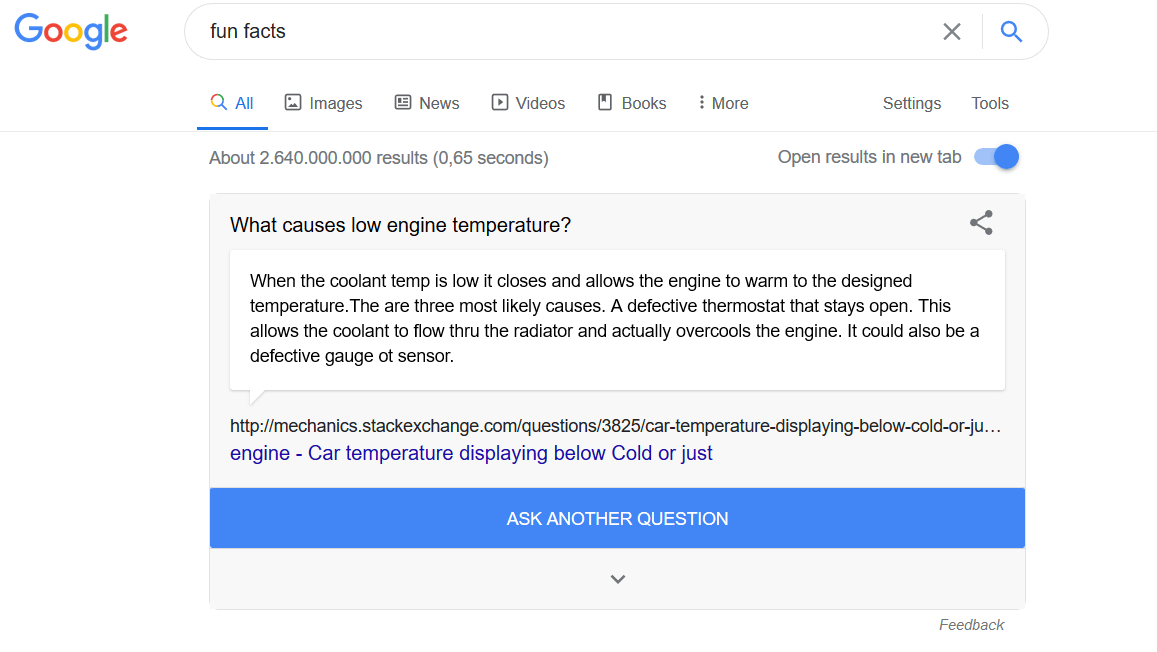The image depicts a Google search page with a search query for "fun facts" displayed. The interface includes familiar elements such as the "All", "Images", "News", "Videos", "Books", and "More" filters below the search bar, along with "Settings" and "Tools" options on the right. The search results indicate approximately 2,640,000 results found in 0.65 seconds, with an option to open results in a new tab, marked by a blue checkbox.

One highlighted result addresses the question, "What causes low engine temperature?" The explanation suggests that low engine temperature can be caused by a defective thermostat that remains open, allowing continuous coolant flow through the radiator and overcooling the engine. Other potential causes include a defective gauge or sensor. The result is sourced from Mechanics.StackExchange.com, with a clickable link that reads "Engine-car, temperature, display, below cold". At the bottom of the snippet, there is an option to ask additional questions for further information.